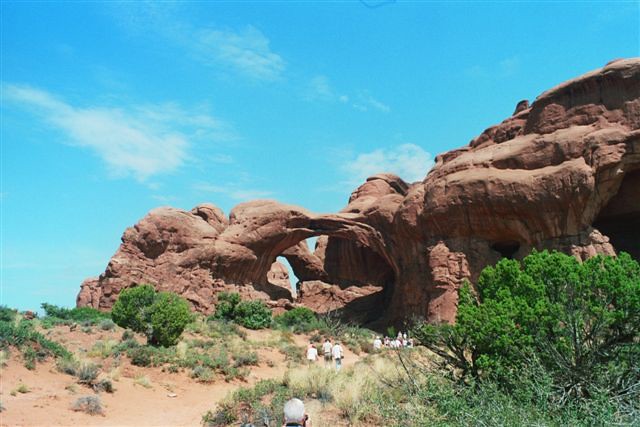In this detailed photograph set in a desert or dry area during the day, a group of around ten people is walking toward a series of towering, red-brown cliffs with diverse shapes, including a prominent natural bridge. The sky above is a vibrant blue, dotted with a few white, wispy clouds. In the foreground, a man's head topped with a gray hat and a tall green bush are visible against the sandy, light brown soil interspersed with smaller bushes. Mid-ground, three individuals in white shirts walk with their backs to the camera, while a blurry group of seven stands at the base of the imposing rock formations. A green, bushy tree can be spotted at the lower edge of the cliffs, partially blue from the shadows, amidst the scattered desert vegetation. The photograph captures the rugged beauty and vastness of the landscape, highlighting the human scale against the monumental natural structures.